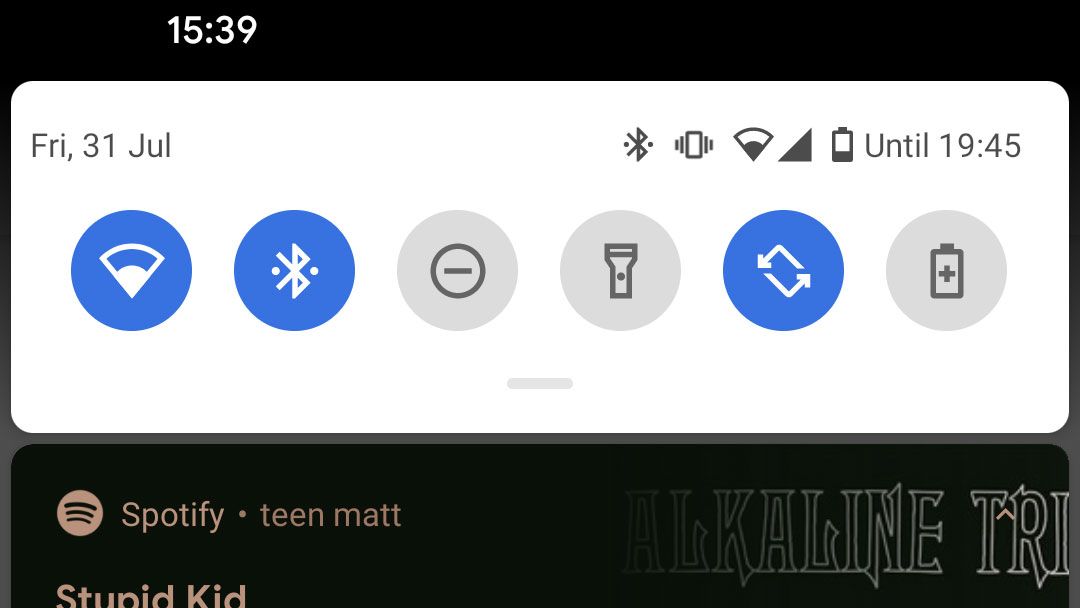The image depicts the upper portion of a smartphone screenshot with a black background. In the top left corner, the time is displayed as "15:39" in white text. Adjacent to it is a large white box. On the left side of this box, the date "Friday, July 31st" is prominently shown, while on the right side, there is a time span indicated as "Until 19:45."

To the far right corner of the display, there are several status icons: a nearly depleted battery icon, a triangular alert symbol, an internet connectivity symbol, a phone icon flanked by lines on either side, and a Bluetooth icon.

Below this section, there are a series of circular icons arranged horizontally:
1. A blue circle featuring a white Wi-Fi symbol.
2. A blue circle with a white Bluetooth symbol.
3. A gray circle with a smaller circle inside it, crossed by a line, indicating a "Do Not Disturb" mode.
4. Another gray circle displaying a flashlight icon.
5. A blue circle with two arrows arranged in a box shape, representing data synchronization.
6. A gray circle with a black battery symbol.

Beneath these icons, there is text that reads: "Spotify Teen Matt, stupid kid," suggesting a Spotify account or playlist title.